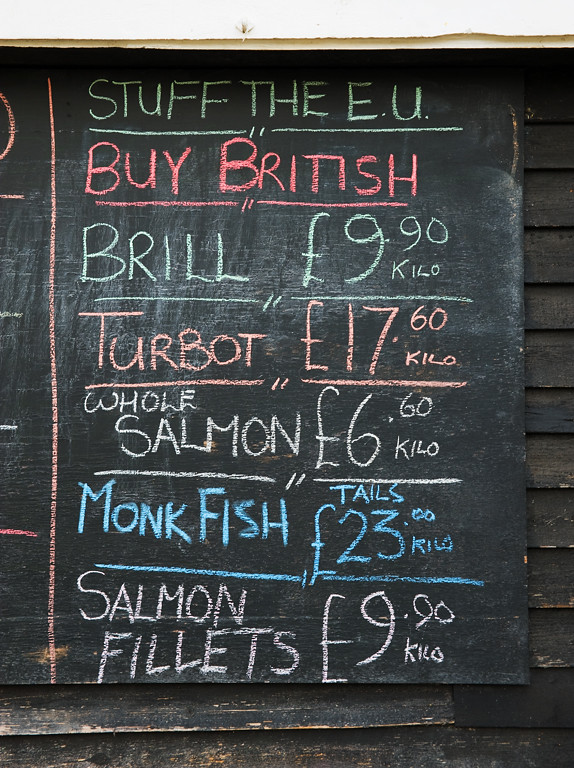The photograph captures a rectangular, well-used chalkboard sign leaning against a building with weathered, black-painted wooden siding. The sign lists various fish prices in colorful chalk, each entry underlined in the same hue. At the top, in green chalk, it reads "Stuff the EU," and beneath it, highlighted in red chalk, "Buy British." The detailed pricings are as follows: "Brill" at 9.90 euros per kilo in light blue, "Turbots" at 17.60 euros per kilo in pink, "Whole Salmon" at 6.60 euros per kilo in white, "Monkfish Tails" at 23.00 euros per kilo in blue, and "Salmon Fillets" at 9.90 euros per kilo in white. Each price is prefixed with a euro symbol.